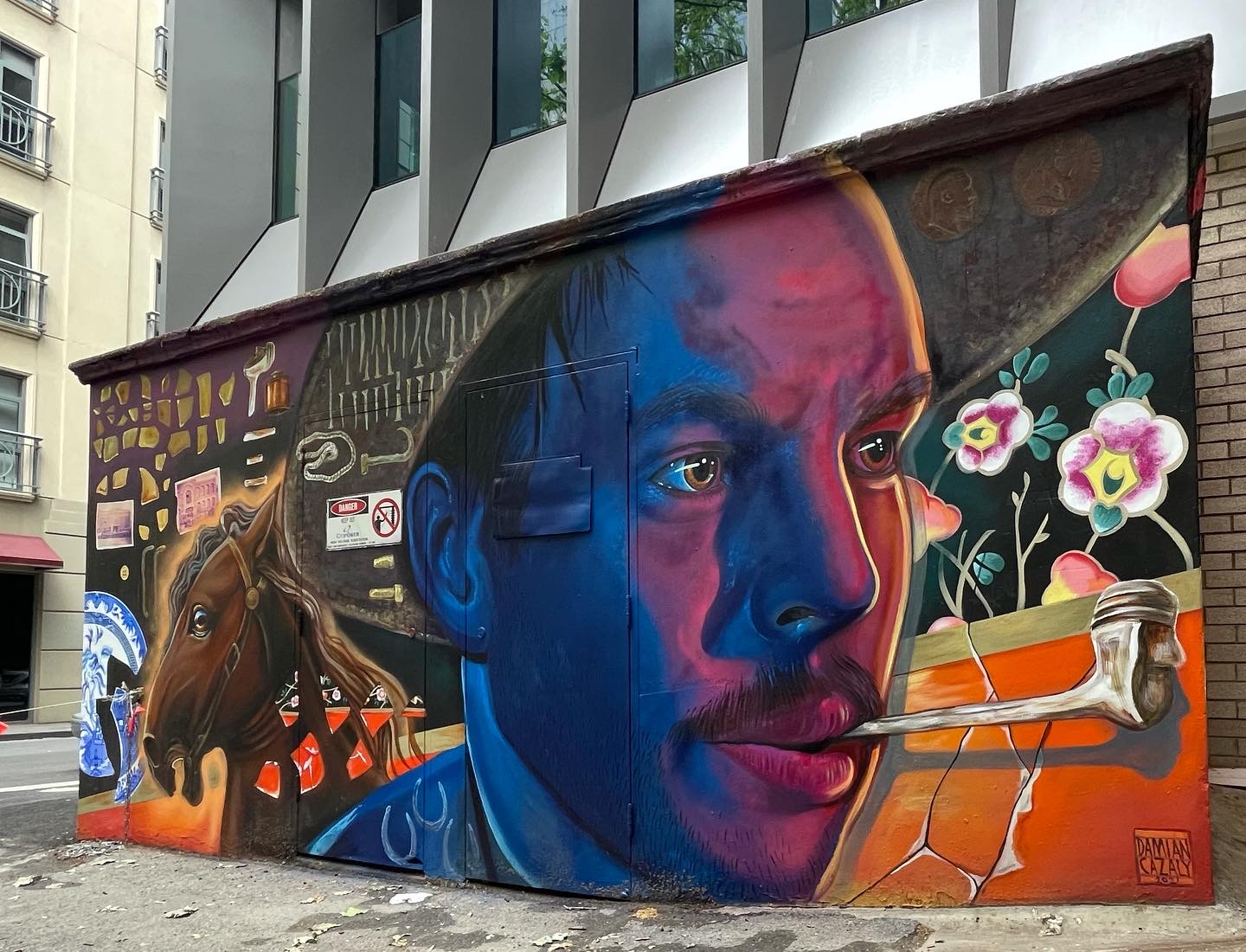This photograph captures an outdoor mural painted prominently on a structure that appears to extend onto a sidewalk, with a larger building featuring a series of windows in the background. Dominating the mural is a surreal, geometric depiction of a man’s face, rendered in striking detail with contrasting hues: the left side in cool blues and the right side in warm reddish tones, accented by a gold or yellow highlight. The man is adorned with a large cowboy hat and a mustache, and he holds a white pipe in his mouth, which intriguingly ends in a smaller face. Although no smoke emanates from the pipe, a backdrop of flowers blooms behind it. To the left of the man’s face, a brown horse is depicted with an open mouth, as if expressing shock. Above the horse hover a series of symbols or fragmented shards. The horse’s head is encircled by a yellow glow and painted next to it is a broken glass plate. The mural’s vivid and varied motifs create an intricate tapestry of textures and colors.